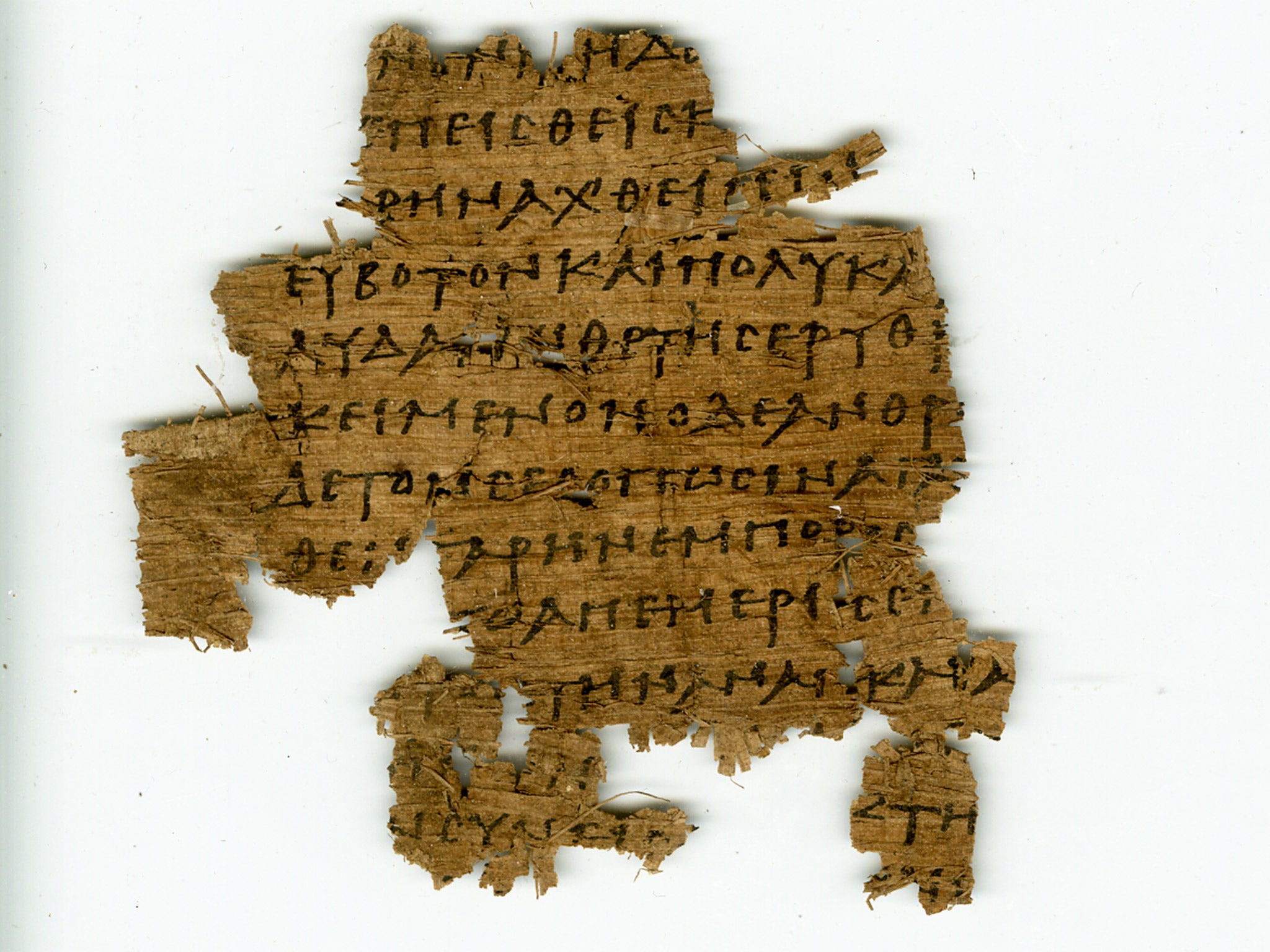The image depicts an ancient artifact resembling a piece of bark, possibly an artifact from a physical anthropology dig. It is brown and appears quite brittle, with a ragged and worn surface that suggests it was torn from a larger piece. The texture is reminiscent of old, fragile paper or wooden fibers. Scattered across the surface is a sequence of letters that seem unfamiliar, with some resembling Roman characters but not forming any recognizable English words. These letters are black and appear to be handwritten, perhaps with a quill. The overall condition of the material is delicate, with crinkled edges and significant wear, hinting that it might break if handled. This artifact, set against a white background, gives the impression of being centuries old, resembling an antiquated message lost over time.